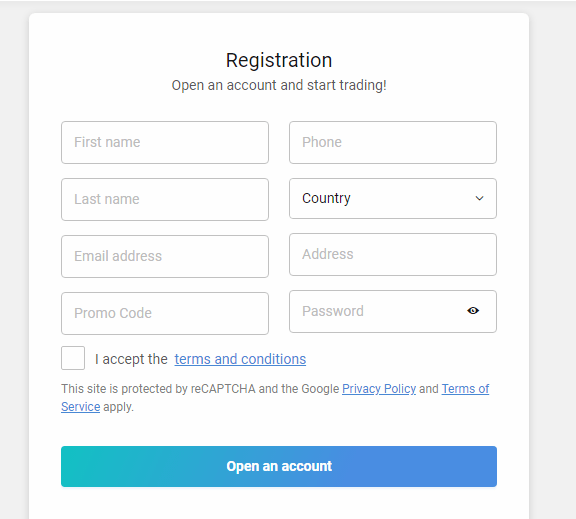**Detailed Caption:**

The image depicts a minimalistic registration interface for a website or app dedicated to account creation, featuring a predominantly white central form area surrounded by a light gray border. This user-friendly design ensures all essential fields are clearly presented. 

At the top center of the form, a bolded "Registration" header is prominently displayed, immediately followed by "Open Accounts.html" in smaller text. 

The form consists of two evenly divided columns, each containing four input fields. On the left column:
1. **First Name:** A text input field.
2. **Last Name:** A text input field.
3. **Email Address:** A text input field.
4. **Troll Code:** A text input field, which appears to be a unique identifier or promotional code.

On the right column:
1. **Phone Number:** A text input field.
2. **Country:** A dropdown menu allowing the user to select their country.
3. **Address:** A text input field.
4. **Password:** A text input field with an eye icon, enabling users to toggle the visibility of their password input.

Beneath these input fields, there's a checkbox labeled "Accept the Terms and Conditions," which users must check to proceed with registration. Just below this checkbox is a disclaimer: "This site is protected by reCAPTCHA and the Google Privacy Policy and Terms of Service apply," with "Privacy Policy" and "Terms of Service" underlined to indicate hyperlinks.

Finally, at the bottom of the form, there is a large, attention-grabbing button in a blue-green gradient labeled "Open Accounts," inviting users to submit their information and create an account.